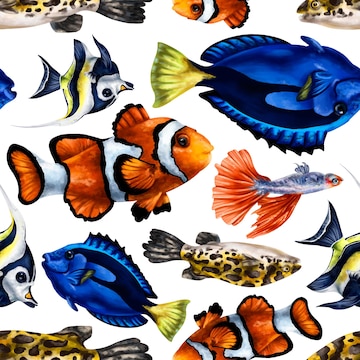This image, which appears to be an excerpt from a book or magazine and has a slightly vintage aesthetic, showcases a hand-drawn collection of colorful fish against a white background. The fish exhibit a range of intricate designs and semi-realistic details. Among the various species illustrated, there are blue fish with yellow fins, orange and white striped clownfish, and fish with distinctive leopard-print patterns. 

Some of the fish, like the close-up of a clownfish, are swimming right side up, while others, like a larger blue tang, are floating upside down. Notably, many of the fish, including the vividly depicted moorish idols and blue tangs, face from left to right, although a few face the opposite direction. The image's composition also gives the impression of being a section cut off from a larger piece. The vivid colors and the dynamic orientations of the fish contribute to a visually engaging artwork that captures the diversity and beauty one might see in a fish tank or zoo exhibit.